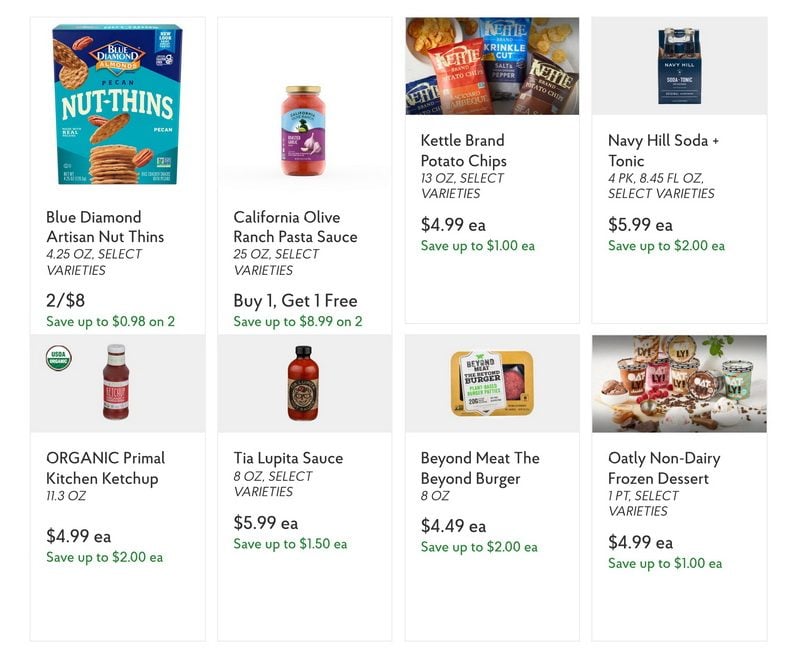The image displays eight distinct food items, each detailed in individual rectangular boxes. 

1. Blue Diamond Artisan Nut Thins: 4.25 ounces, available in select varieties, with a promotion of two for $8.
2. California Olive Ranch Pasta Sauce: On a buy one, get one free offer.
3. Kettle Brand Potato Chips: Priced at $4.99 each.
4. Navy Hill Soda Plus Tonic: Available for $5.99 each.
5. Organic Primal Kitchen Ketchup: 11.3 ounces, priced at $4.99 each.
6. Tia Lupita Sauce: 8 ounces in select varieties, priced at $5.99 each.
7. Beyond Meat Beyond Burger: Priced at $4.49 each.
8. Oatly Non-Dairy Frozen Dessert: One pint, in select varieties, priced at $4.99 each.

Beneath these product descriptions, potential savings for each item are highlighted in green, featuring phrases like "save up to 98 cents on two" and "save up to $8.99 on two." The rest of the text, which provides details on size, quantity, and prices, is displayed in black lettering.